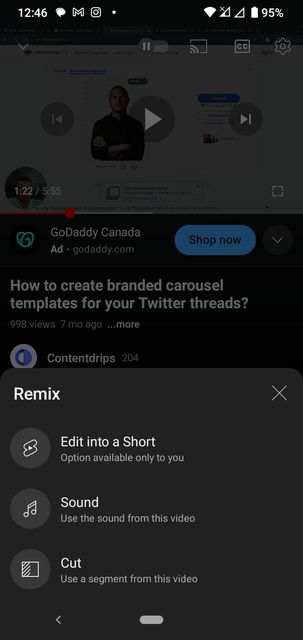A screenshot captured from a smartphone displays a predominantly black background. In the top-left corner, the time reads 12:46, followed by a letter 'M' and a camera icon. The battery indicator on the top-right shows a 95% charge. Below, a grayed-out video occupies the central section, featuring a person against a white background. Standard video controls like a play button, and forward/backward buttons are visible over the video.

Beneath the video, an advertisement for "Go Daddy Canada" with the web address "GoDaddy.com" is displayed, accompanied by a blue "Shop Now" button. The text, "How to Create Branded Carousel Templates for Your Twitter Threads," appears below, suggesting the video's topic.

At the bottom, a gray interface box contains a white "Remix" label in the upper left, an 'X' to the right, and three options underneath: "Edit into a Short," "Sound" (with a music note icon indicating the option to use the video's sound), and "Cut" (for using a segment from the video).